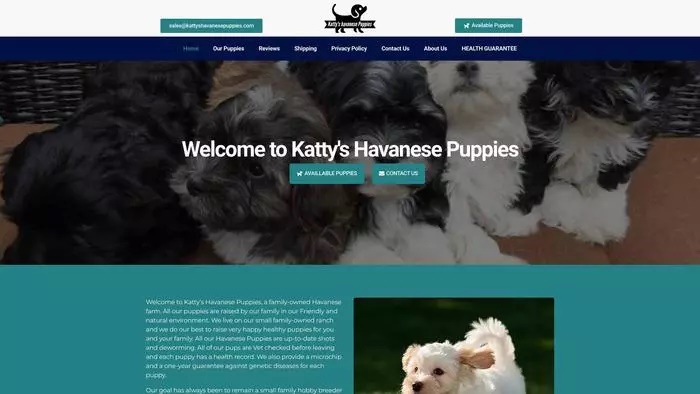This is a detailed screenshot of a desktop website for Caddy's Puppies. At the top center of the screen, there's a logo featuring a dog accompanied by text. On either side of the logo, white text appears on a teal background. This entire section is set on a white bar. Below, a blue navigation bar displays various option buttons including Home, Our Puppies, Reviews, Shipping, Privacy Policy, Contact Us, About Us, and Health Guarantee, all in white text on the blue background.

The next section features a slightly grayed-out image of three puppies lying huddled together on a table with a wicker background, presumably showcasing the puppies from the business. Above this image, white text reads "Welcome to Caddy's, Have Any Puppies." Below, there are two teal buttons with white text labeled "Available Puppies" and "Contact Us."

Further down, the background changes to solid teal featuring a block of text in the center, next to a photo of a small white dog running against a dark, slightly green background. Both the text and the image appear truncated, suggesting the need to scroll further to view the complete content.